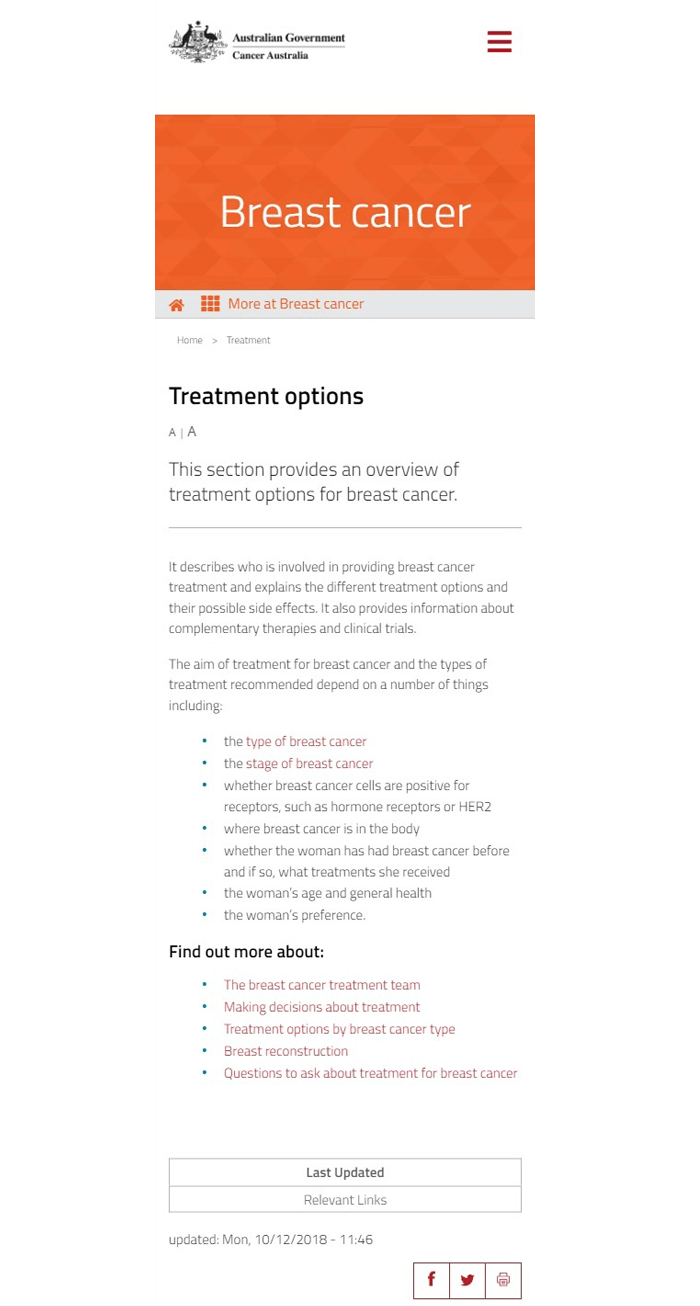Screenshot of a mobile website from the Australian Government's Cancer Australia:

- At the top left, the Australian Government logo is displayed in black, accompanied by what appears to be a family crest.
- On the right side of the header, there is an orange menu button.
- Directly beneath the header, an orange banner with white text reads "Breast Cancer," followed by a subheading "Treatment Options."
- Below this, there are small and large text buttons for easy navigation.
- The section provides an informative introduction stating, "This section provides an overview of treatment options for breast cancer."
- A horizontal line divider separates this introduction from the detailed content below.
- The main text passage discusses the key professionals involved in breast cancer treatment and elaborates on the various treatment options available.
- Following the passage, a bullet-point list appears, highlighting essential considerations such as the type and stage of breast cancer.
- At the bottom of the screenshot, there is a section titled "Find out more about," potentially leading to more detailed information or resources.